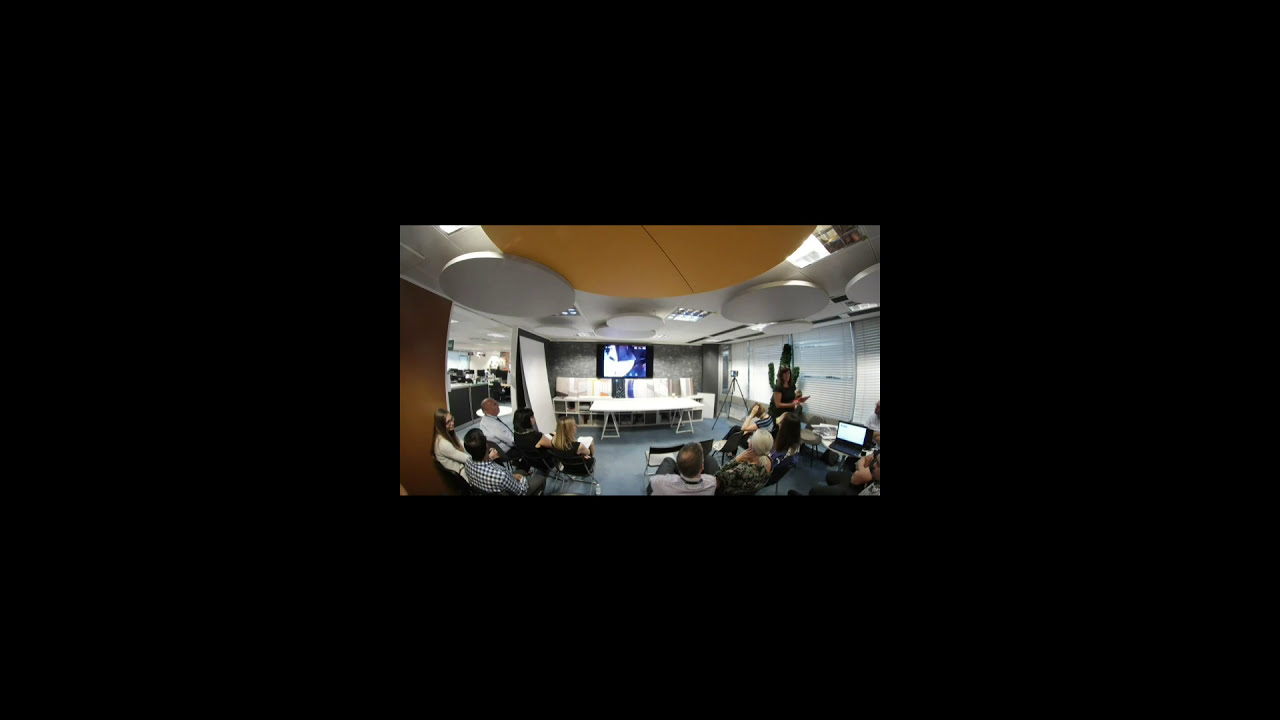This detailed color photograph, presented in a small, inset panoramic format against a black background, captures the interior of a classroom or conference room. In the forefront, a few rows of seated individuals face away from the viewer, directing their attention towards the front of the room. Here, a white fold-out table is positioned, adorned with various colorful posters and framed against a black pull-down lecture screen displaying a blue and white image. A woman, dressed in black with brown hair, stands on the right side of the room. The ceiling is notable for its engaging design, featuring an orange circular pattern with white disks that adds a corporate and neat aesthetic. At the very top, a yellowish-orange half-disk is partially visible. The left side of the image reveals a brown wall and windows that provide a glimpse into another area of the building. This room appears highly organized, suitable for either educational or conference purposes.